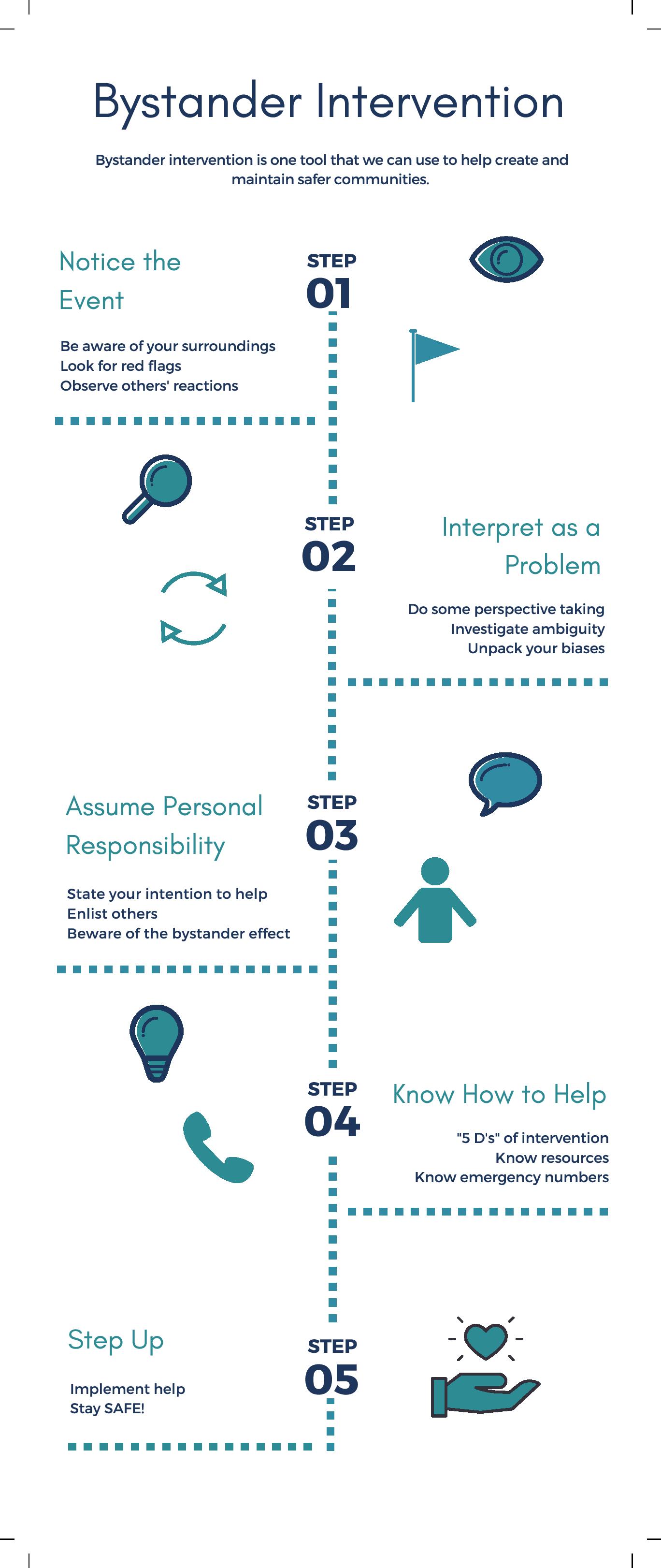The image is a detailed vertical poster illustrating a five-step process for bystander intervention, designed to create and maintain safer communities. At the top, the title "Bystander Intervention" is prominently displayed in black font. Below the title, steps are organized sequentially along a central line, connected by blue dotted squares.

Step 1, situated on the left, instructs to "Notice the Event," emphasizing the importance of being aware of surroundings and looking for red flags. This step is illustrated with an icon of an eye and a flag in blue and black.

Step 2, positioned on the right, advises to "Interpret as a Problem," encouraging perspective taking and the recognition of biases. This step is represented by a magnifying glass and two arrows curved in a circle.

Step 3, found on the left, tells the reader to "Assume Personal Responsibility," highlighting the necessity of stating one's intention to help and enlisting others, while being aware of the bystander effect. An icon of a person and a speech bubble illustrates this step.

Step 4, appearing on the right, is to "Know How to Help," explaining the five Ds of intervention and the importance of knowing emergency numbers and resources. This step is depicted with a telephone and a light bulb.

Step 5, located at the bottom left, prompts to "Step Up" and implement the help while ensuring one's safety. This final step is symbolized by an icon of an upward-facing hand with a heart above it.

Overall, the poster's design is elongated and rectangular, with all text in a coherent blue font and accompanied by simple blue and black illustrations that reinforce each step visually.